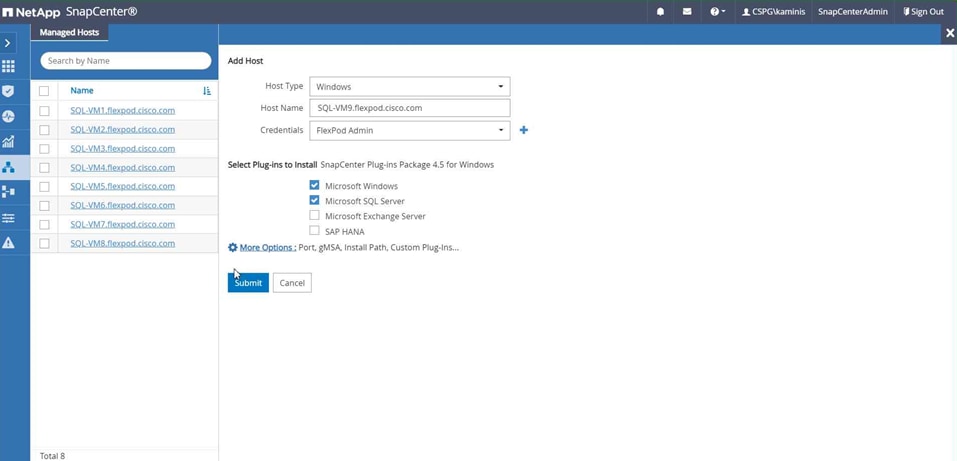The image depicts a webpage interface for NetApp SnapCenter. On the left side of the screen, there is a vertical navigation bar with a teal blue background. The navigation bar features various icons including an arrow pointing to the right, and a 3x3 grid of squares, followed by a shield with a check mark, a circle with a heartbeat line, a graph with an arrow pointing upwards, a standard share button, a different type of share button, a circle with an unknown icon, and a triangle with an exclamation mark. Among these, the highlighted icon is related to managed hosts.

To the right of this navigation bar is the main content area. At the top of this area, there is a search bar labeled "Search by Name" for data entry. Below the search bar is a list of eight items. Each item in the list has a checkbox to its left and a uniform format for the naming convention, starting with "SOL-VM" followed by a number ranging from 1 to 8 and ending with "flexpod.cisco.com". None of the checkboxes are currently selected. The background of the items in the list is blue, and each line is separated for clear distinction.